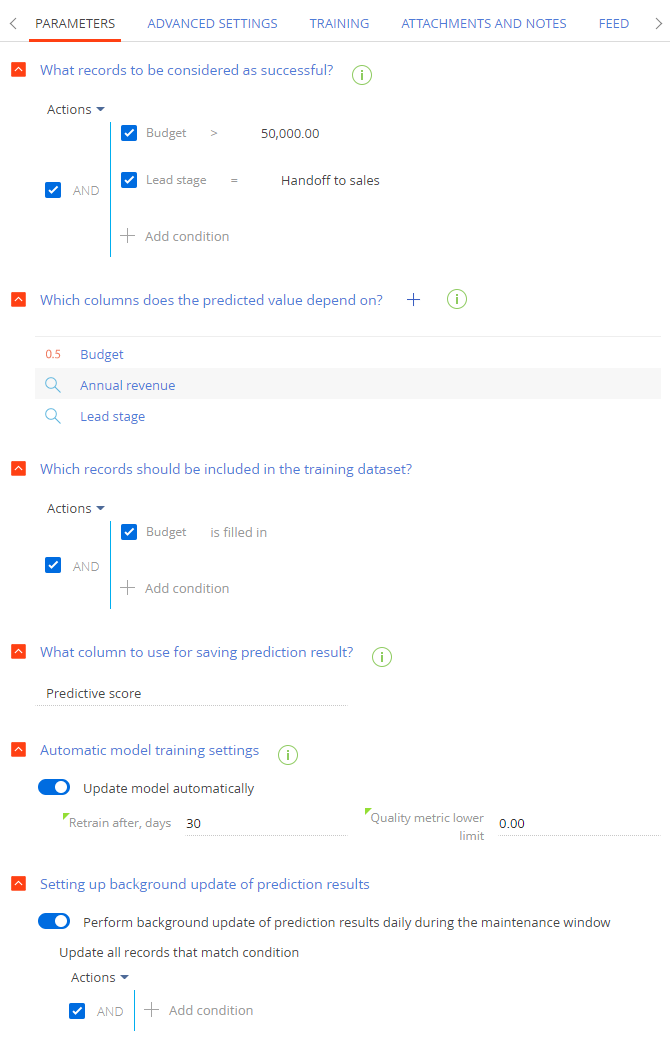This detailed image depicts a comprehensive webpage interface designed for managing predictive model training and settings. The interface is segmented into multiple sections and boxes, each dedicated to specific functionalities. 

1. **Parameters Box:**
   - Provides options to define various parameters required for model training.

2. **Advanced Settings Box:**
   - Allows customization of detailed configurations beyond the default settings.

3. **Training Box:**
   - Includes settings related to the training process of the predictive model.

4. **Attachments and Notes Box:**
   - Facilitates the addition of supporting documents and notes for reference.

5. **Feed Box:**
   - Displays updates and notifications about ongoing processes.

6. **Records Considered Successful:**
   - Specifies criteria for what records are deemed successful.

7. **Actions Section:**
   - Contains actionable items, including a checked `Budget` box set to $50,000 and a condition for `Lead Stage` equal to "handoff to sales."
   - Features an "Add Condition" button with a plus sign for adding new criteria.

8. **Predicted Value Dependencies:**
   - Lists columns impacting the predicted values including Budget (0.5), Annual Revenue, and Lead Stage, each accompanied by a magnifying glass icon for further inspection.

9. **Training Data Set Inclusion:**
   - Details which records should be part of the training data set, with the `Budget` box checked.
   - Provides an option to add new conditions and specifies the column for saving prediction results as "Predictive Score."

10. **Automatic Model Training Settings:**
    - Includes options to update the model automatically, with a checkbox for retraining after a set number of days, currently set to 30 days.
    - Sets a quality metric lower limit at 0.00.
    - Enables background updates of prediction results daily during the maintenance window, applied to all records matching specified conditions.

Each section is thoughtfully organized, providing a user-friendly interface for configuring and managing predictive models efficiently.